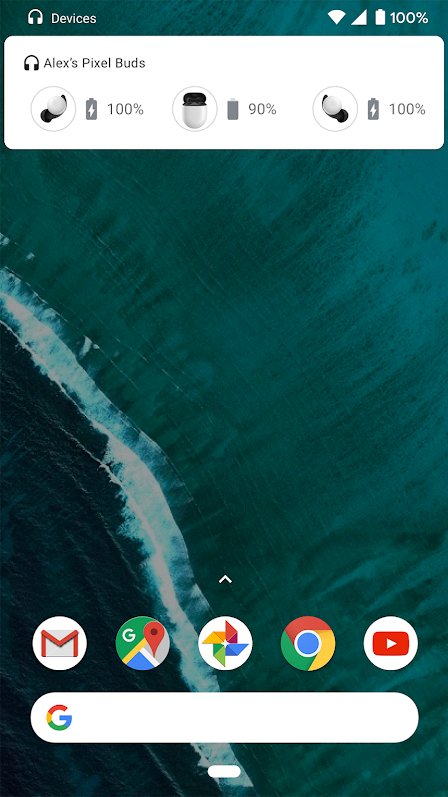The image features a greenish-blue background with a pair of headphones icon and the text "Devices" alongside a "100% battery" indicator at the top. Below this, there is a white box labeled "Alex's Pixel Buds" with icons showing "100% battery" and "90% battery". Central to the image, there are arranged pictures of the ocean. Towards the bottom-middle of the screen, an upward-pointing arrow is displayed. Below this arrow, there are several distinct icons in circular white backgrounds including: 

1. An envelope with a big red "M" on it (likely representing Gmail).
2. A multi-colored "G" (green, yellow, white, blue, and gray) with a small red pin (possibly Google Maps).
3. A multicolored windmill-like icon in blue, green, yellow, and red (possibly representing Google Photos).
4. A Google Chrome icon with yellow, green, and red segments, containing a blue circle inside.

Further down, a white circle contains a red box with a right arrow (likely representing YouTube). At the bottom of the screen is a search box featuring the multi-colored Google "G" in red, yellow, green, and blue, accompanied by a small white circle.